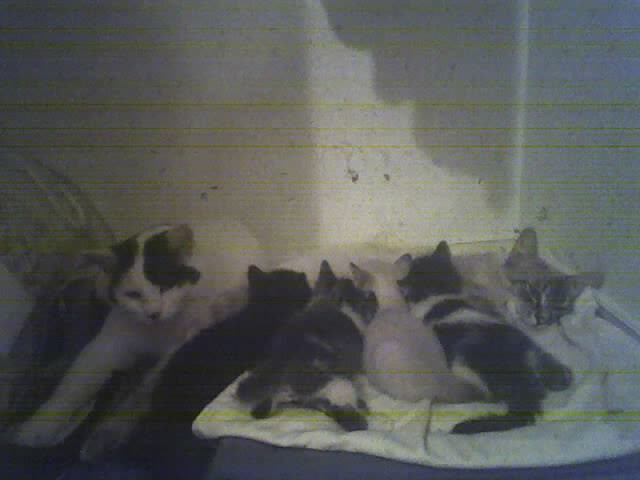The photograph captures a heartwarming scene of feline family life with a mother and father cat, along with their four kittens, nestled on a white towel in a room bathed in soft sunlight. The image, predominantly in shades of black, white, and gray, appears weathered with yellow horizontal lines, giving it a nostalgic, almost vintage feel. The mother cat, a gray tabby, lies contentedly on her side with her kittens nursing from her. The kittens, with their backs turned towards the camera, come in various colors: one solid black, two black and white, and one cream-colored. At the mother's side, the father cat, mostly white with black markings around his head and a distinctive black dot on his nose, lounges protectively. Both adult cats appear relaxed, with their eyes directed towards the camera. The background showcases a white wall, partly illuminated by sunlight from a window, casting a shadow that suggests the presence of a curtain. The scene, though grainy and somewhat blurred, eloquently captures the tender and intimate moment of the cat family.